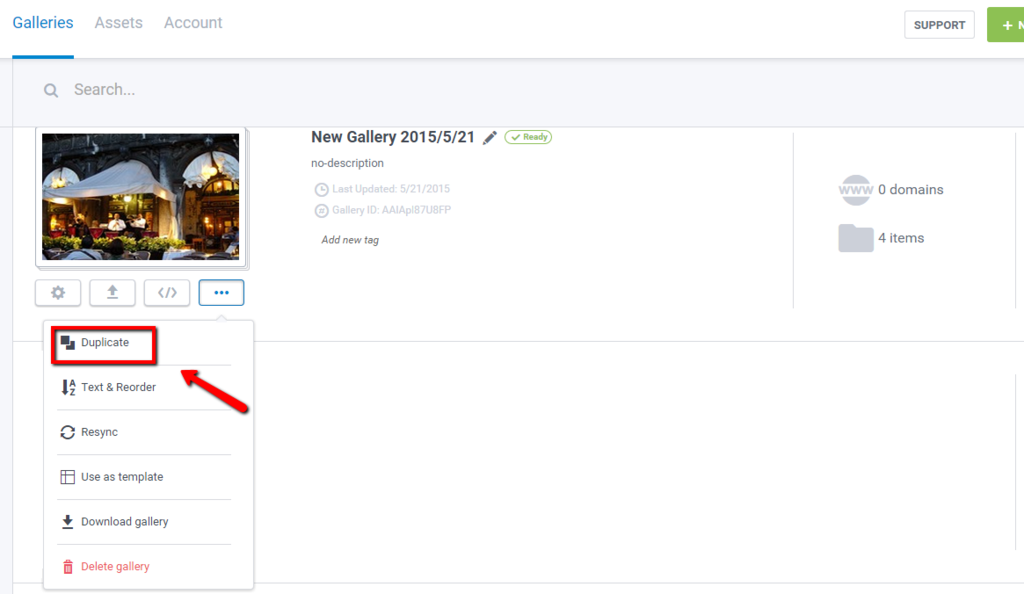This is a cropped screenshot from the Galleries section of the Juxtapose app by Syncopa. The app is designed for creating and managing media galleries, including images, videos, and other files. The background of the interface is predominantly white, giving it a clean look.

In the top left corner of the main section, there is a thumbnail of a photo. Below the photo thumbnail, a vertical row of four small, gray-outlined boxes is present. The first box features a cogwheel icon at its center, likely representing settings. The second box has an upward-pointing arrow, possibly for uploading files. The third box displays arrows pointing left and right, suggesting it is used for scrolling through the gallery images. The last box, located at the bottom, is a menu button, which is currently selected and outlined in blue.

Upon selection of the menu button, a small panel opens up with a list of options: Duplicate, Text and Reorder, Resync, Use a Template, Download Gallery, and Delete Gallery. The 'Duplicate' option is highlighted, indicated by a red box edited around it. A red arrow points from the bottom right towards the 'Duplicate' setting, drawing attention to it.